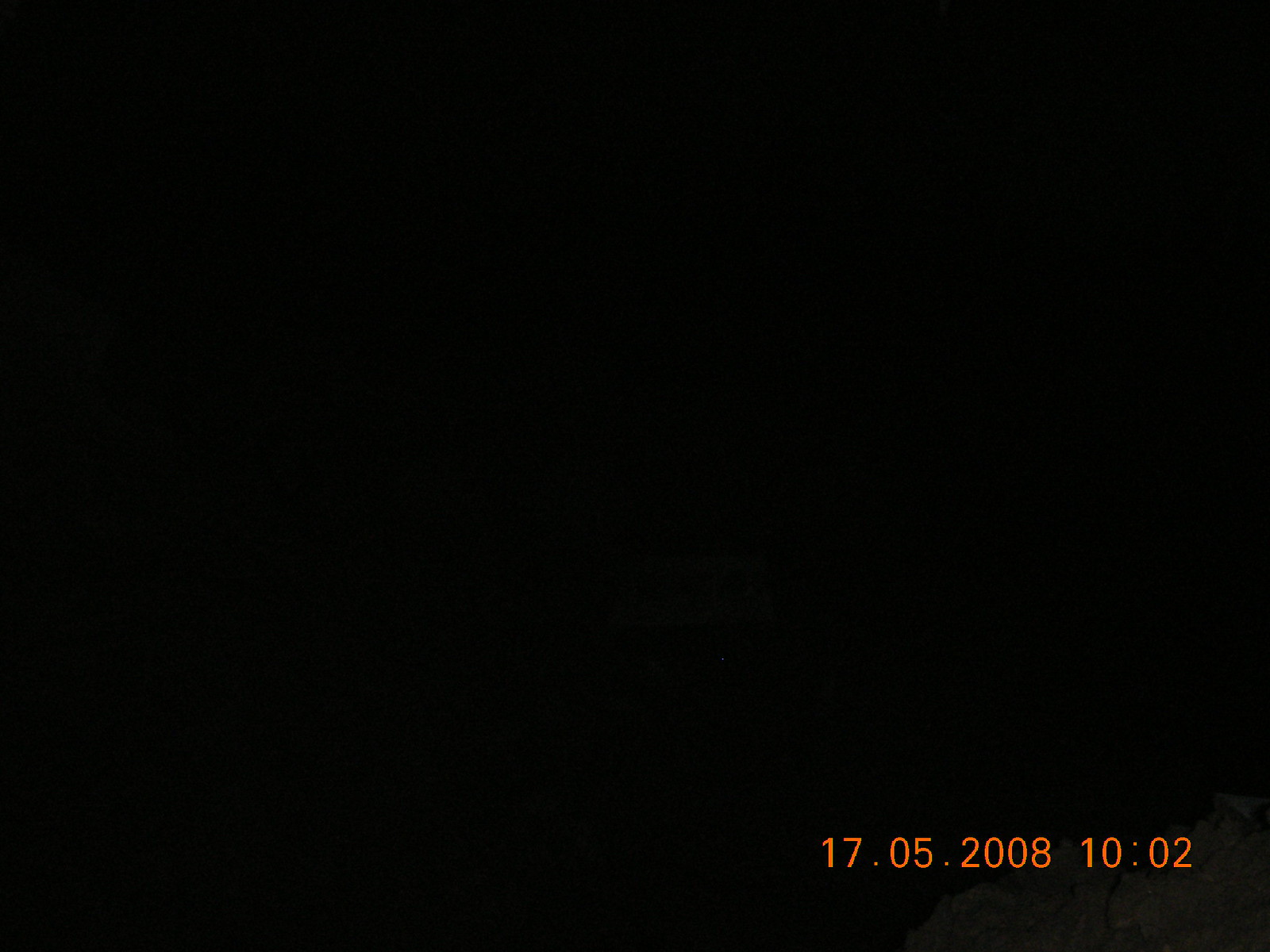A photo shrouded in complete darkness, with no discernible objects or features visible, occupies the frame. The only identifiable element is an orange timestamp located in the bottom left corner, marking the date and time as May 17, 2008, at 10:02 p.m. Beyond this single glowing detail, the image remains an impenetrable void, offering no clues to its subject or setting, leaving the viewer with an enigmatic sense of mystery and absence.